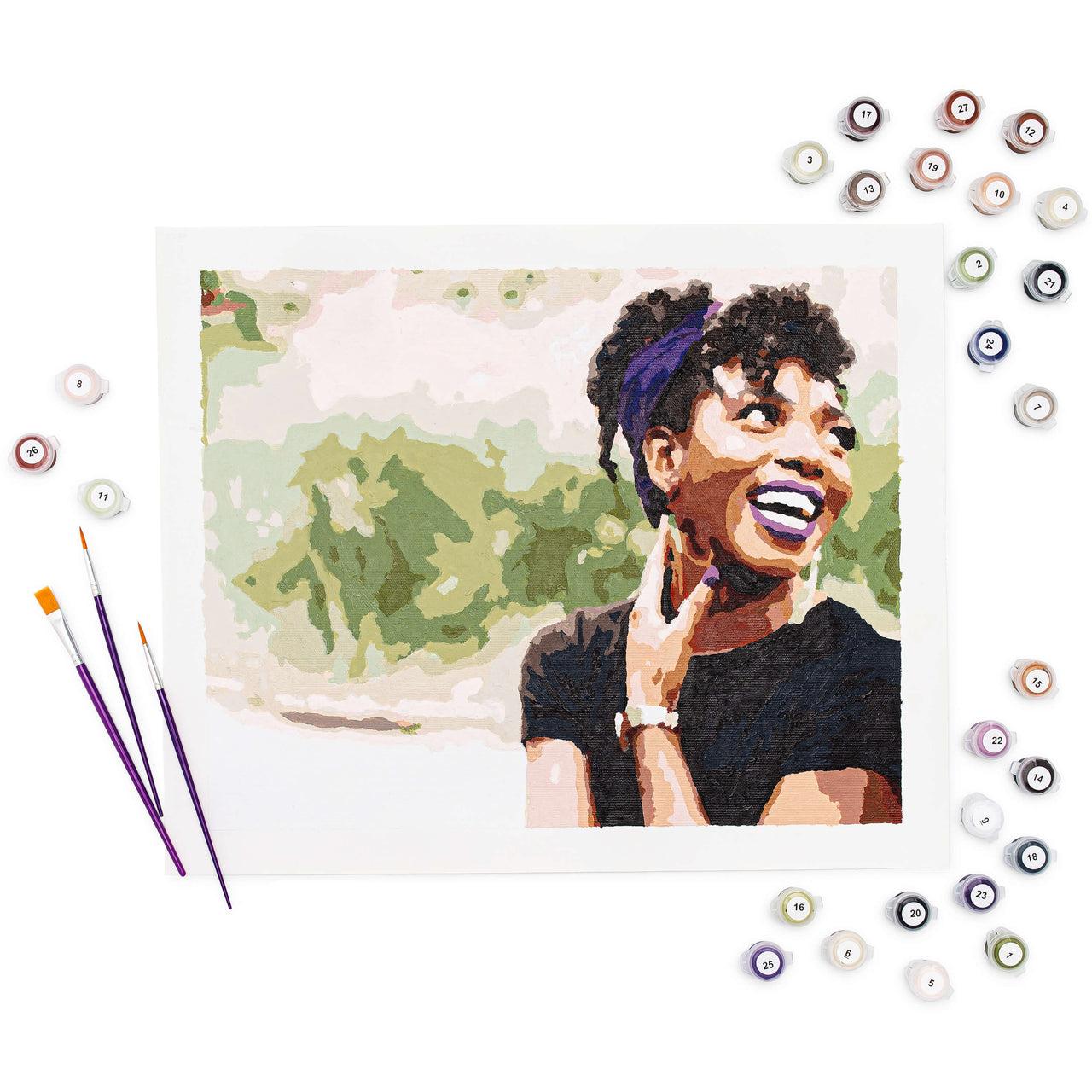The image depicts a vibrant watercolor painting of a young black woman with a deeply radiant smile. She is portrayed with a head of black hair embellished with a purple scarf or ribbon. Her joyous expression is accentuated by her purple lips and purple nail varnish. The woman is seen wearing a black T-shirt and a watch on her left wrist, her right hand gently touching her neck. The background features an abstract nature scene with elements of vegetation, likely trees and hedges, although they lack detailed definition. Surrounding the main picture are several paint cups and three paintbrushes of varying widths. The paintbrushes have brown tips, silver middles, and purple handles. Additionally, there are scattered miniature pots of paint, each marked with numbers that symbolize different colors used in the painting process. This artistic composition is quite abstract, utilizing a limited color palette yet effectively conveying a sense of contentment and joy.